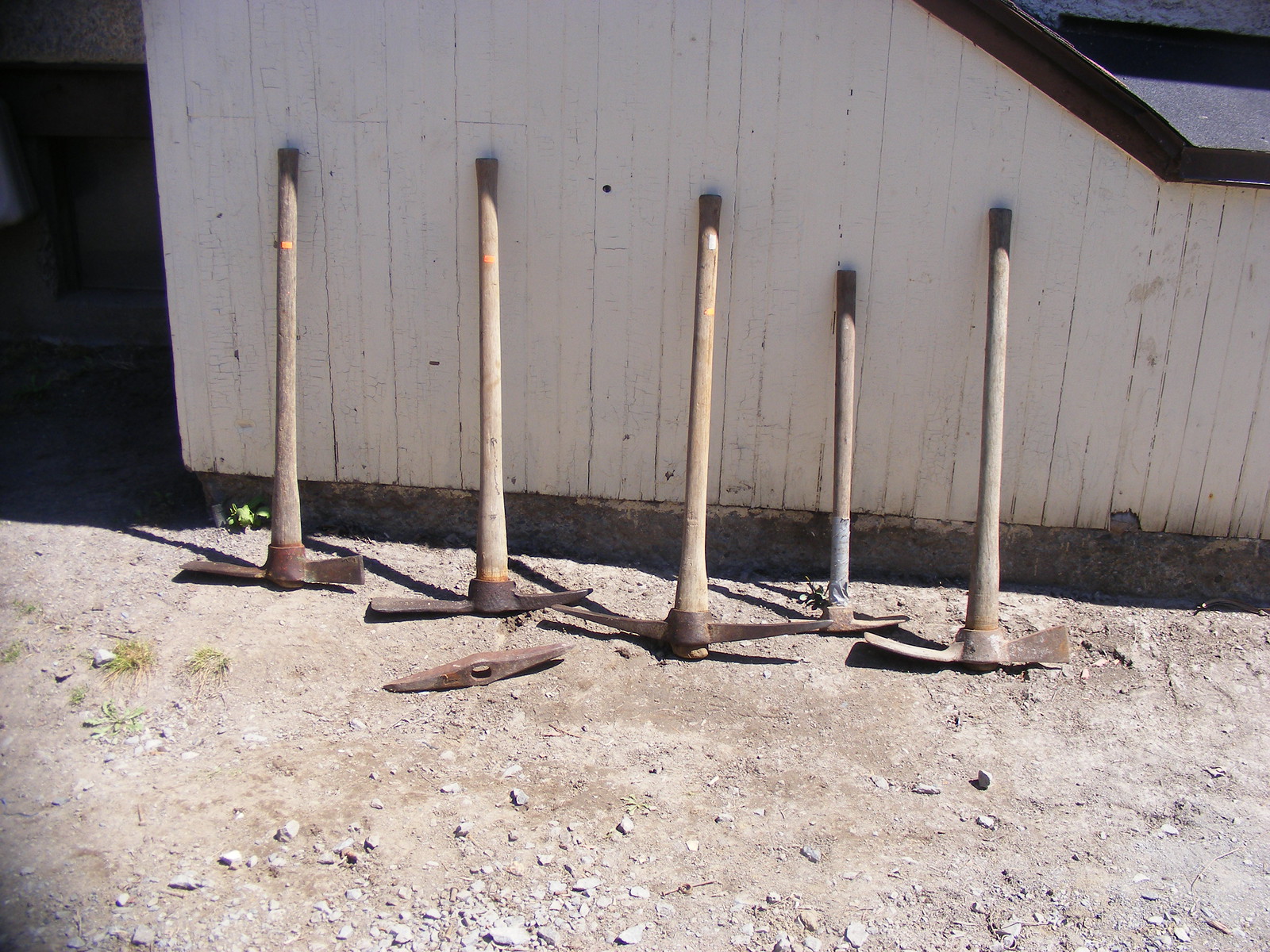The photograph captures a collection of five weathered pickaxes, along with a lone pickaxe blade without a handle, arranged outdoors on a rocky, sandy dirt ground. The pickaxes are propped up against a white wooden building with dark brown trim and a sloping structure. Each pickaxe features a sturdy, round wooden handle that has been worn smooth over time. Notably, the metal heads of the pickaxes are slightly rusty, reflecting their age and frequent use. A couple of the handles display bright orange dots, adding a splash of color to the otherwise muted scene. The ground is scruffy, with patches of green grass and scrappy weeds poking through. Amid the assortment, one pickaxe appears to have been repaired, evidenced by tape around its top part. The ambiance suggests a sense of history and rugged utility, with the tools showing signs of their long service.